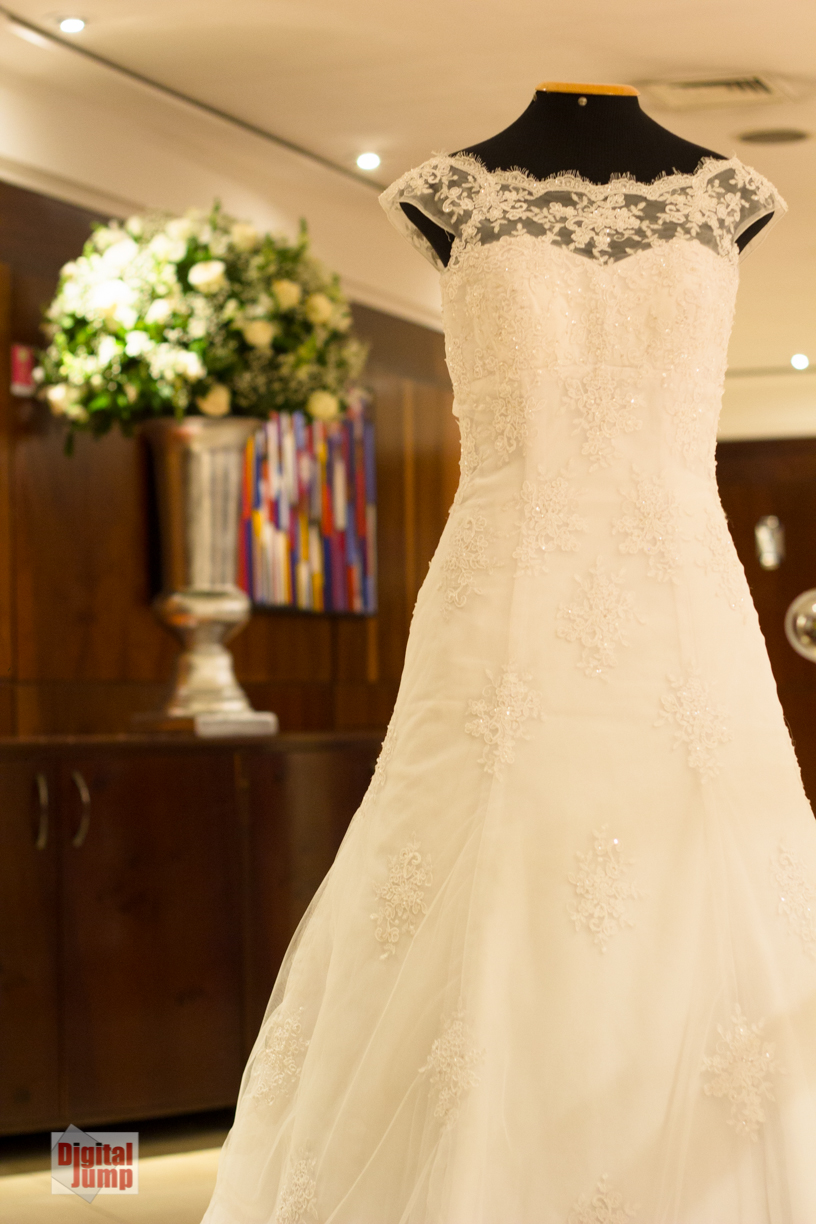The photograph captures an elegant, white bridal dress displayed on a headless and armless black mannequin, positioned to the center-right. This sleeveless wedding dress features a lacy upper section with delicate decorative patterns reminiscent of snowflakes, and it flares out towards the bottom, taking up a significant portion of the bottom half of the image. The mannequin, devoid of arms and head, prominently showcases the dress.

In the background, slightly out of focus due to the depth of field, there are mahogany brown cabinets adorned with metal handles. Positioned atop these cabinets is a large, silver vase filled with a lush bouquet of white flowers interspersed with green sprigs, possibly roses or light yellow blooms. The background also includes a brown wooden wall with blurry, vertical stripes of white, red, blue, and yellow artwork. A plain white ceiling with recessed lighting illuminates the scene. 

In the very lower left-hand corner of the image, there is a small watermark on a white background with red text stating "A Digital Jump," suggesting the photograph may have been taken in a store or showroom specifically for wedding dresses.